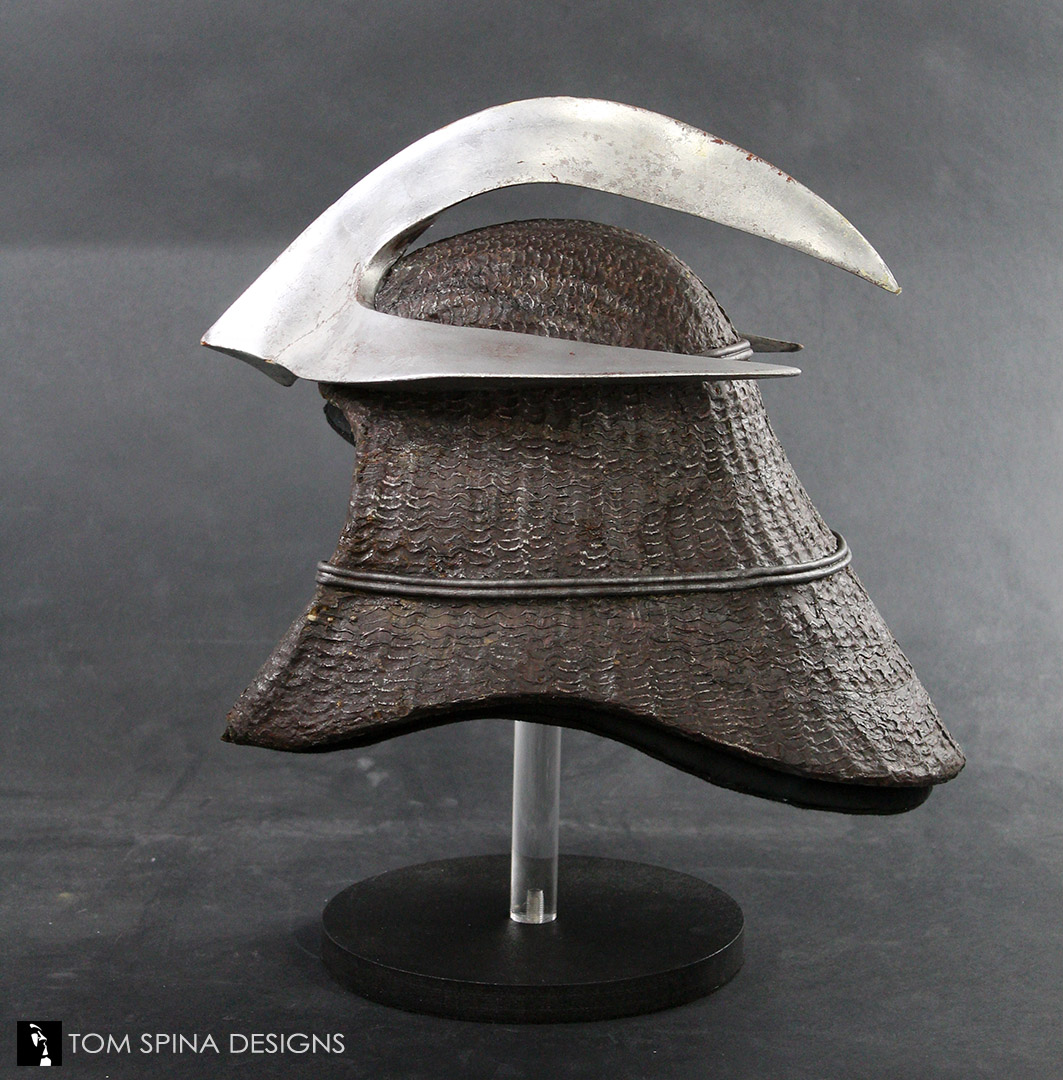The photograph captures a striking black-and-white image, possibly with sepia undertones, featuring a detailed sculptural helmet. The image is horizontally short and set against a light gray, mottled background that highlights the central object. In the bottom-left corner, the photograph bears the logo and text "Tom Spina Designs."

The helmet, which rests on a black wooden disc about a centimeter high, is set atop a plastic tube that serves as its stand. The main body of the helmet is textured metal with intricate carvings resembling fish scales, and it encompasses the head, extending almost to the shoulders and slightly forward in front of the chin. A ridge runs around its center, adding to the detail and structure.

Atop the helmet is a prominent, shiny, polished metal piece, sharp and dagger-like, which arcs over the top of the helmet, creating an imposing and almost weapon-like appearance. The piece connects at the front and features wings that stretch around the sides, giving the helmet an abstract yet medieval, possibly Celtic or Viking aesthetic. The overall impression is both historical and stunningly artistic.